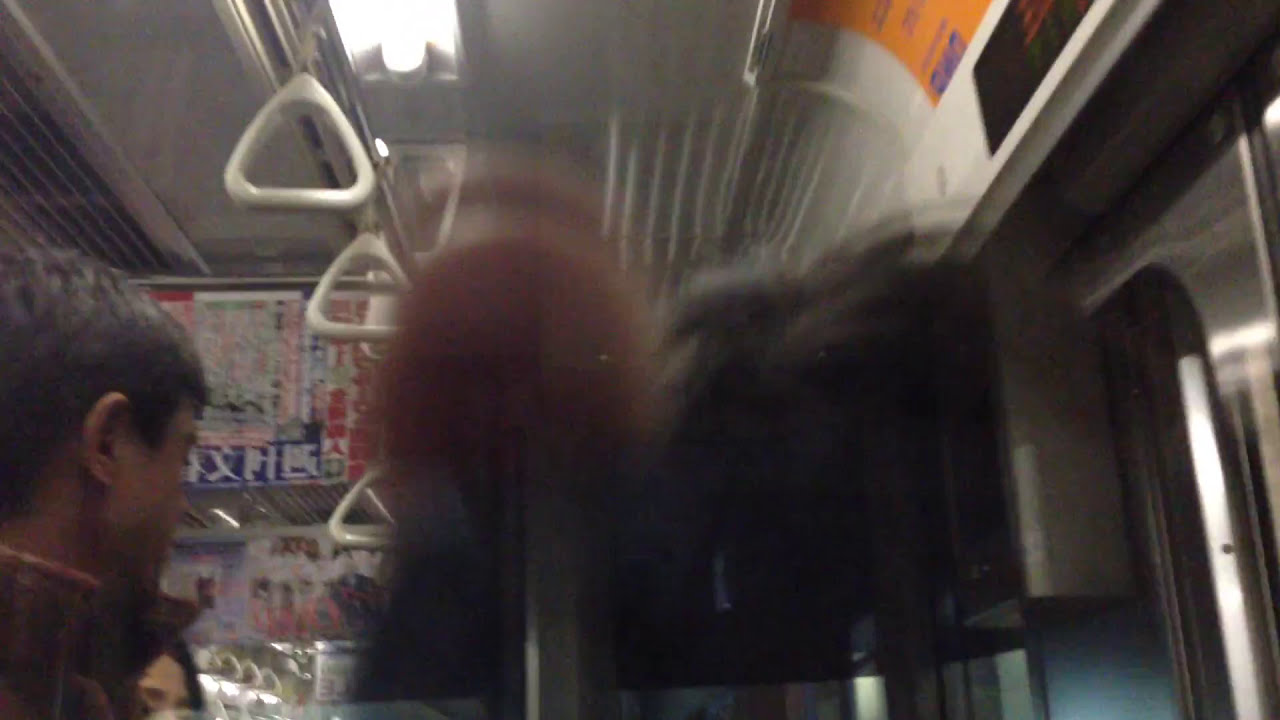In the image, an Asian male and female are positioned in the bottom left corner, their bodies slightly angled as if awaiting their exit from a fast-moving subway. The man, with black hair, is dressed in a red and yellow plaid jacket, while the woman's face is partially obscured. Above them, white triangular handholds dangle from a ceiling rail, and the car is illuminated by bright white lights. To the right, a mechanical door with unreadable signage suggests the exit route. A colorful poster featuring Asian script is prominently displayed in the foreground, adding to the bustling atmosphere of what appears to be an Asian subway setting. The scene is filled with vibrant hues, including black, brown, red, orange, blue, pink, purple, and white, highlighting the daily commute in a crowded urban environment.